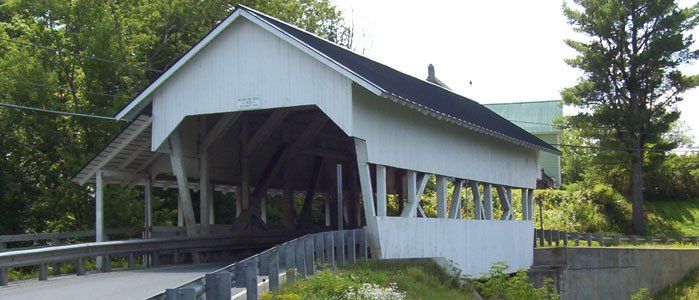This is a daytime photograph of a picturesque, short covered bridge with a blend of quaint and classic design elements. The bridge features white wooden siding with dark gray or blue angled roofs, reminiscent of a typical house, situated over what appears to be a stone or concrete base. In the lower left-hand corner, a road with metal guardrails leads into the bridge and veers to the right. The bridge’s sides have beams that allow light to filter through, revealing that the interior is not entirely dark. Adjacent to the bridge is a brown pedestrian walkway separated by guardrails.

Flanking the bridge on the left side and in the lower left-hand corner are lush green trees and a backdrop of bushes and grass, interspersed with telephone or electricity poles and wires. On the right side, additional greenery including a large tree and more bushes ascend a small hill. Above, the sky is a bright white, indicative of an overcast day, but sunshine and shadows suggest intermittent clouds. In the distance behind the bridge, part of another white building with a metal roof peeks through the foliage. The scene captures a tranquil, rustic atmosphere with an interplay of natural and man-made elements.